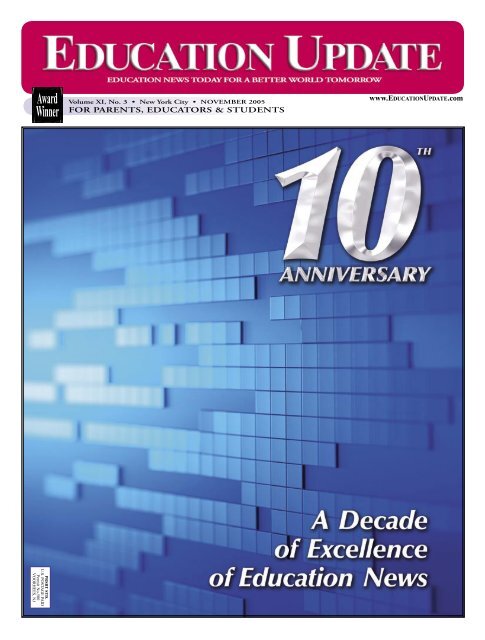The image is a detailed graphic featuring a blue-tinted background composed of small cubes or blocks varying in shades from light blue on the left to the darkest blue on the right, giving a gradient effect. At the top, there is a prominent red rectangle with white text that reads "Education Update," followed by a subhead in a pinkish-red color that states "Education News Today for a Better World Tomorrow." There is a small black box labeled "Award Winner" on the left side underneath the header. To the right, beneath the main title, it says "10th Anniversary: A Decade of Excellence in Education News." Additionally, there is smaller text noting the target audience—parents, educators, and students—and a reference to a web address. In the bottom left corner, a tiny box contains more text that was not clearly legible. The overall design is reminiscent of a book cover, newsletter, or possibly a CD cover with a computer-themed aesthetic.